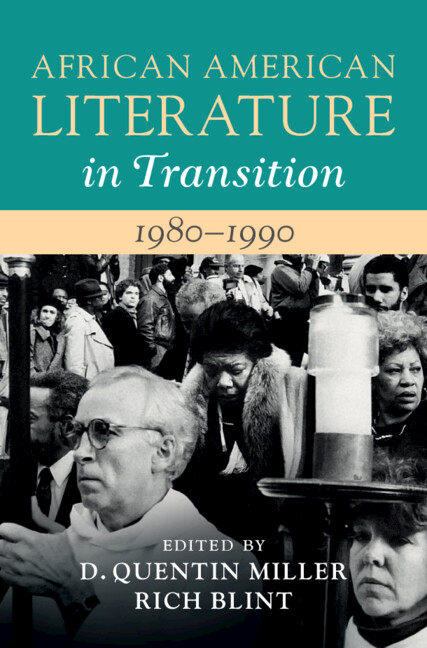This is a detailed description of the cover of the book "African-American Literature in Transition: 1980 to 1990," edited by D. Quentin Miller and Rich Blint. The top portion of the cover features a teal-cyan bar with the title "African-American Literature" written in tan-colored text. Directly below, "In Transition" is inscribed in white. Beneath this, there's a narrow tan (or beige) strip displaying the years "1980 to 1990" in contrasting text. The lower half of the cover showcases a poignant black-and-white photograph capturing a significant moment—a mixture of emotions and cultural settings. In this image, a white man who appears to be a Catholic priest with glasses is holding a candle, possibly part of a larger procession. Beside him, an African-American woman dressed warmly, possibly in a fur coat, looks somber, indicative of mourning. The scene appears to involve multiple individuals, suggesting either a march or a spiritual gathering, though the exact context remains ambiguous. At the very bottom, the editors' names, D. Quentin Miller and Rich Blint, are prominently displayed. This blend of colors, text, and image encapsulates the thematic depth of the transitional period in African-American literature.